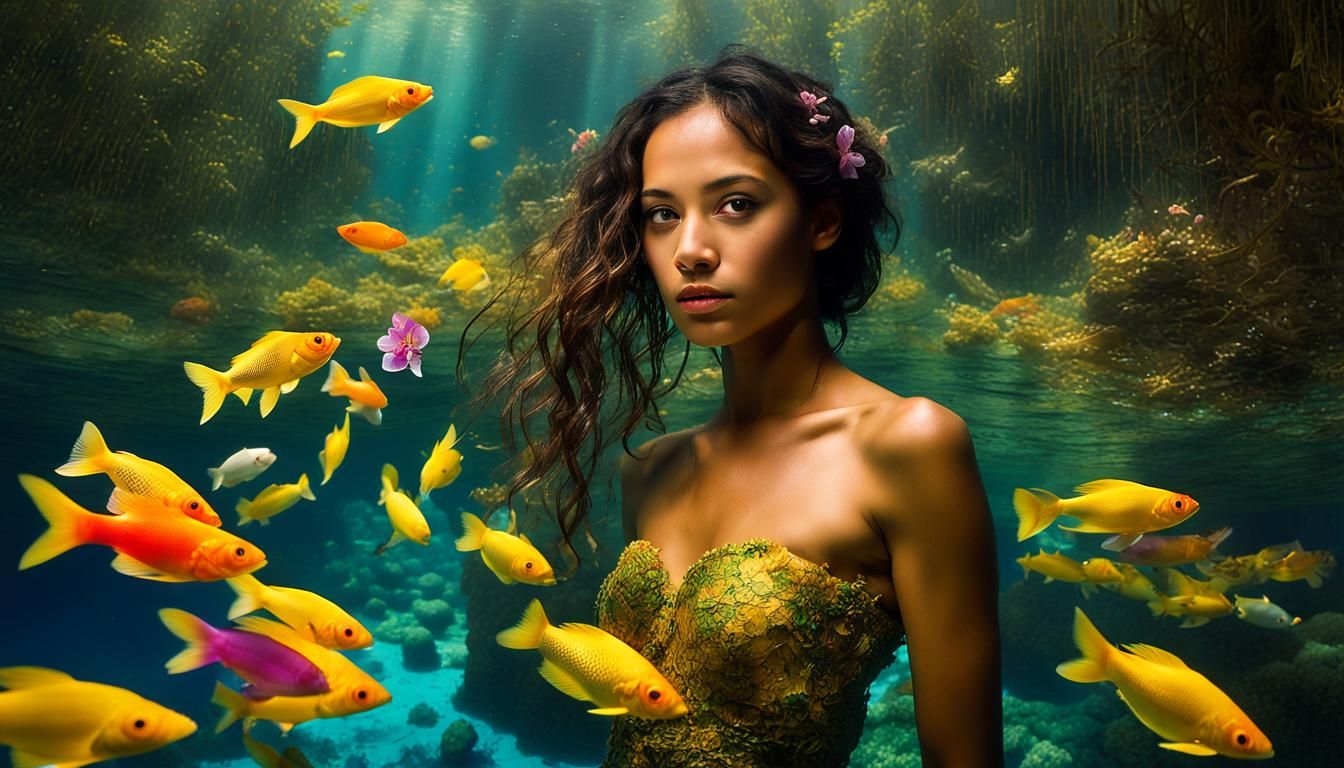The image depicts a surreal, digitally enhanced or AI-generated scene featuring a woman with rich olive-toned skin and long, dark, wavy hair that lightens at the edges. She has curly hair adorned with small purple flowers and is dressed in a garment reminiscent of coral or nature, covering her chest. Positioned at the center of the composition, she gazes directly at the viewer with a blank expression. Surrounding her are gold and yellow fish, seemingly undisturbed by her presence, which enhances the surreal underwater atmosphere. The background showcases underwater vegetation, coral, and light shafts penetrating the water, but the woman herself appears composited onto the scene, evoking a mermaid-like aura. The entire scene blends underwater elements with a dreamlike, otherworldly quality.